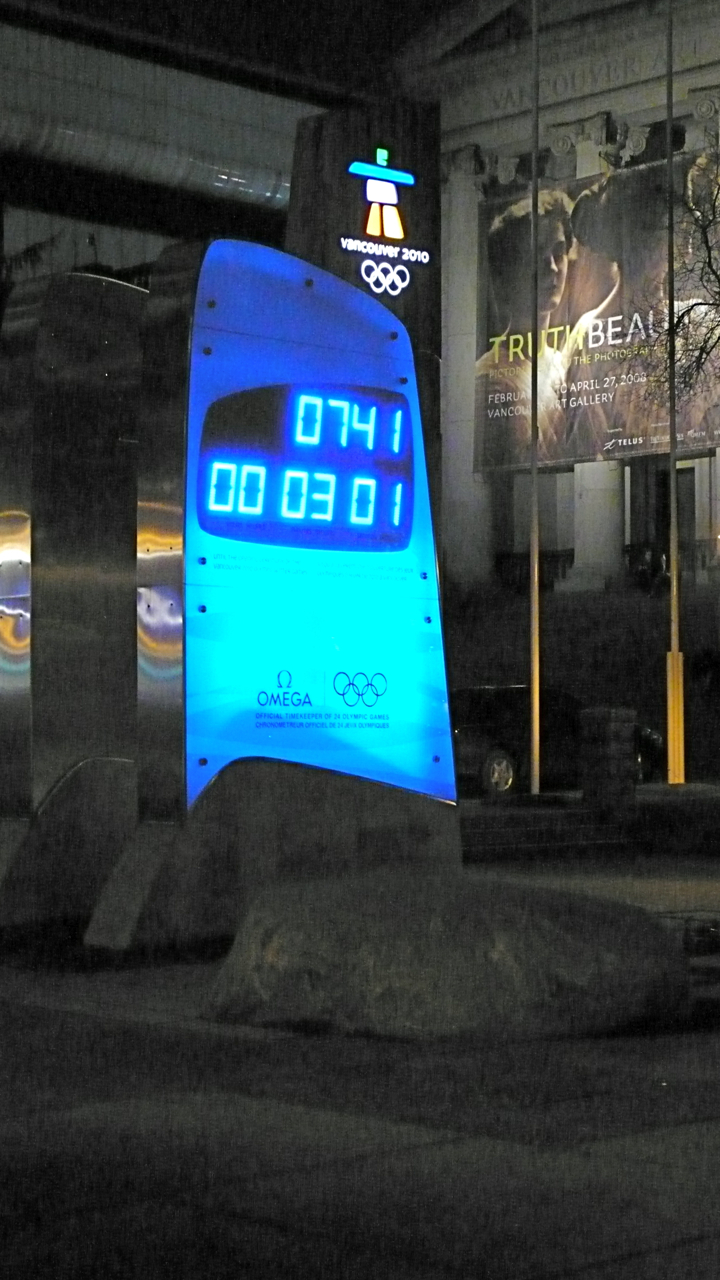Amidst a nighttime urban setting, a strikingly illuminated giant countdown clock stands prominently on a cement platform among some stones. The clock, bathed in a gradient of bright to dark blue from bottom to top, features prominently the "Vancouver 2010" logo along with the iconic interlocking Olympic rings symbol. The brand name "Omega" is also displayed just below the Olympic rings, reinforcing the official timing partnership.

The digital display on the clock reads "0741" and "000301," suggesting it is counting down to or displaying the time as 7:41 AM on March 1st. Adjacent to this Olympic monument, to the right, there's a billboard for the Vancouver Art Gallery featuring an advertisement that includes the partial phrases "Truth Bow" or "Truth Beautiful." The advertisement showcases images of two women dressed in what appears to be Victorian attire, further hinting at an ongoing exhibition.

In the background, the Vancouver Art Gallery is partially visible, confirming the cultural context of the location. Completing the scene, a distant black car with a shiny silver hubcap can be seen, contributing to the urban ambience and depth of the photograph.